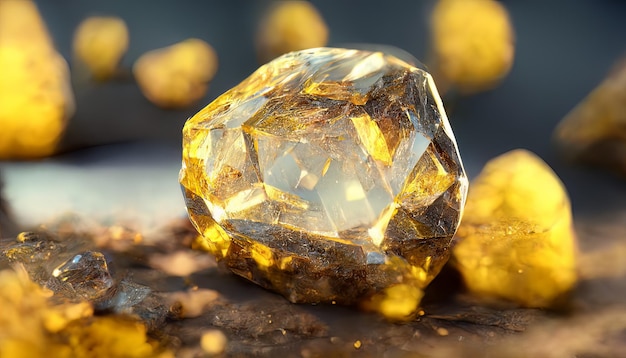A detailed photograph displays a striking yellow gemstone with amber-like highlights set against a brown background. This gemstone, partially translucent and sparkling, occupies the central focus of the image. Off to the right, there is a solid yellow orb, which appears rock-like and non-translucent. Both the gemstone and the orb float against a blurred gray background, where additional yellow gems can be faintly observed. In the bottom left corner, yellow powder, seemingly fragments from the gemstone, lays scattered as if the gem is in the process of being shaped into a jewel. The overall composition of the photograph draws attention to the intricate details and varying states of the yellow gem, from rough to finely cut, emphasizing its transformation.